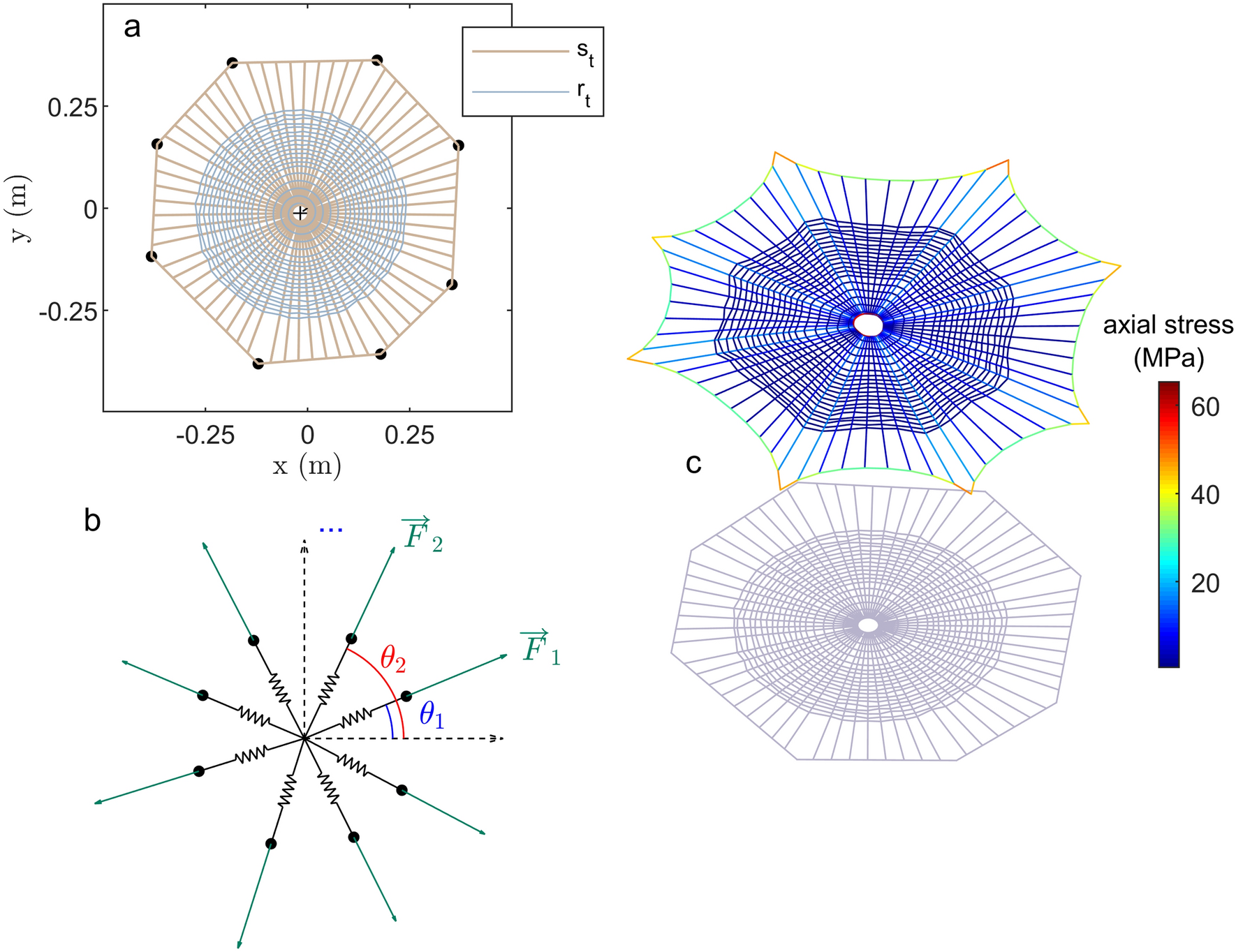The image showcases a series of intricate physics stress graphs on a white background, segmented into three main sections labeled A, B, and C. Each graph displays a spiderweb-like pattern with lines radiating from a central nucleus. The A graph features brown lines, representing spatial data, encapsulated in a black rectangular box. The B graph, distinguished by straight, green lines forming a star-like shape, measures wave features with axes ranging from -0.25 to 0.25 meters and labels indicating B and numerical values. The C graph, predominantly blue and gray, illustrates axial stress with a color gradient bar from 20 MPa (dark blue) to 60 MPa (dark red), positioned on the right side of the image. The shared visual complexity and detailed annotations suggest the image is likely sourced from an advanced physics textbook.